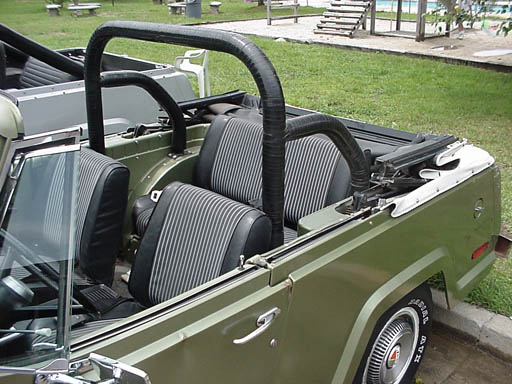This is a highly detailed color photograph taken at a park, capturing a sage green, vintage convertible Jeep from the driver's seat perspective, just past the windshield towards the back end. The vehicle features a tall black roll bar behind the black and white striped leather front seats, with a small bench seat in the rear. The car, with its white-walled tires and old-fashioned silver door handle facing forward, is parked next to a grassy area. In the background, a playground can be seen with its steps and swings, set against a bordered sandy area. The driver's side vent window is open, and the top of the car is down, revealing its elaborate interior. Another similar silver vehicle is partially visible, parked to the right. The photograph is devoid of people and legible writing.